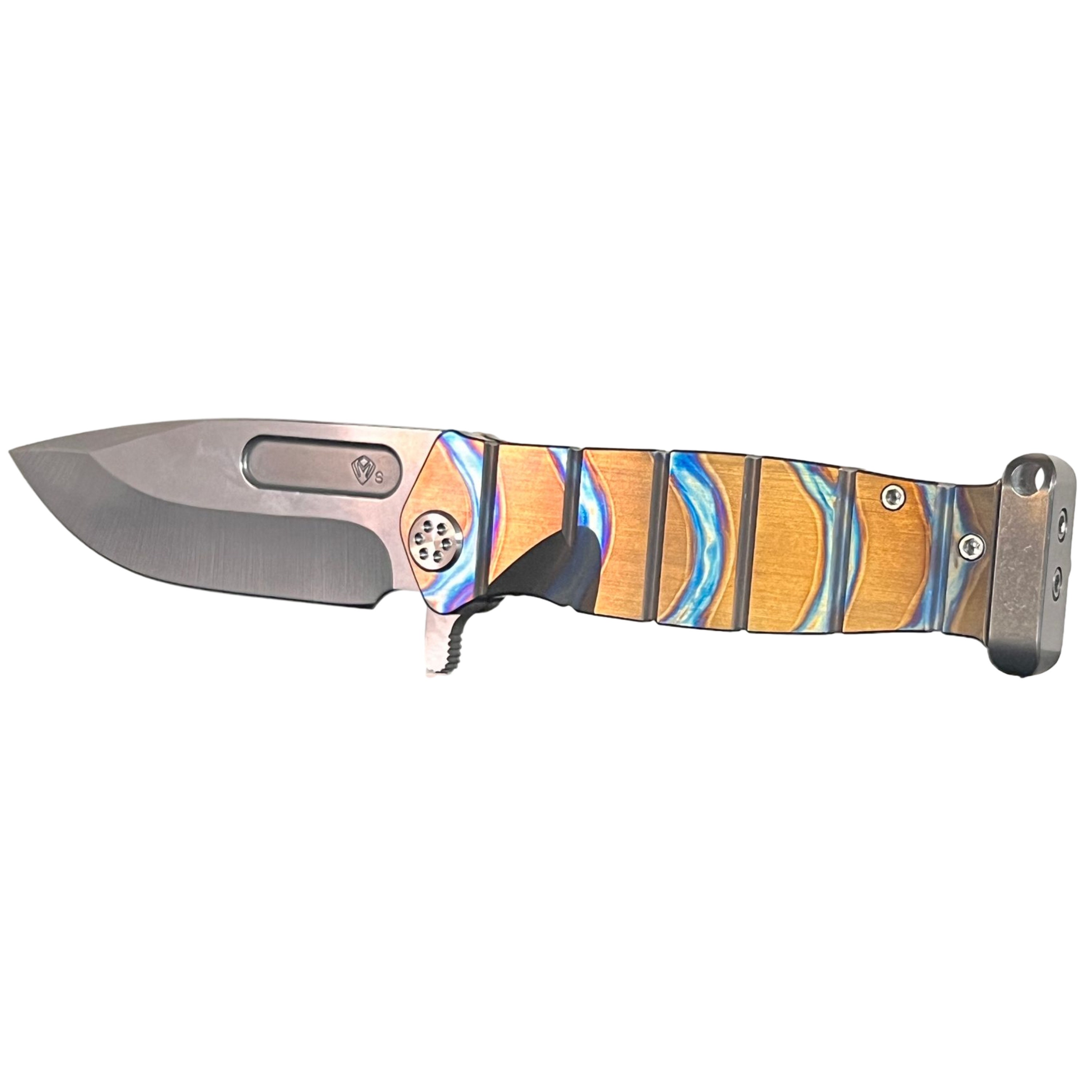A detailed close-up image of an elegant pocket knife, with its grayish-silver blade open and pointing to the left. The blade features a distinctive flat edge on one side and a beveled edge on the other, along with a small, oval cutout near its base. Within this oval, the number "9" is subtly engraved. The knife's handle is beautifully sectioned, exhibiting a rich honey wood color interspersed with blue half-circle accents. The bottom part of the handle incorporates a rounded, dark bronze metal piece, enhancing its aesthetic appeal. Additionally, the lower two sections of the handle are secured by two small, silver screws, offering both functionality and style.